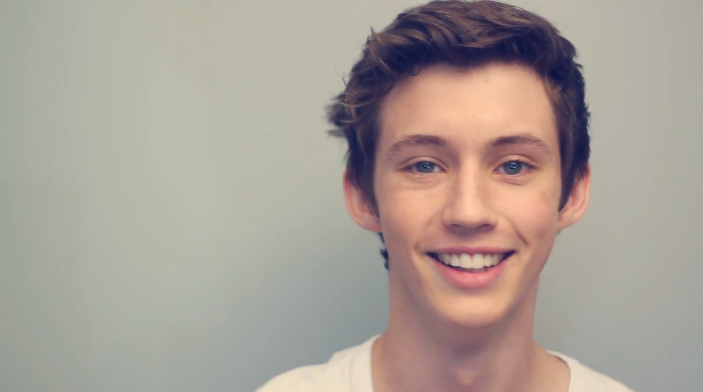This photograph captures a young Caucasian male, likely an older teenager or in his early twenties, shown from the upper shoulders to the top of his head. He wears a white shirt and stands against a plain grey background, which darkens at the edges due to the lighting. His brown hair is of medium length, swept and brushed backward, framing his face attractively. The young man’s expression is cheerful, with a wide smile that exposes his upper row of white teeth. He possesses brown eyes that reflect light, adding depth to his gaze. His head is positioned towards the right side of the photograph, leaving a notable amount of empty space on the left. Subtle shadows cast by the lighting add a touch of dimension to the backdrop. This image appears professional and polished, resembling a headshot potentially used for modeling or advertisements, highlighting his pleasant and approachable demeanor.